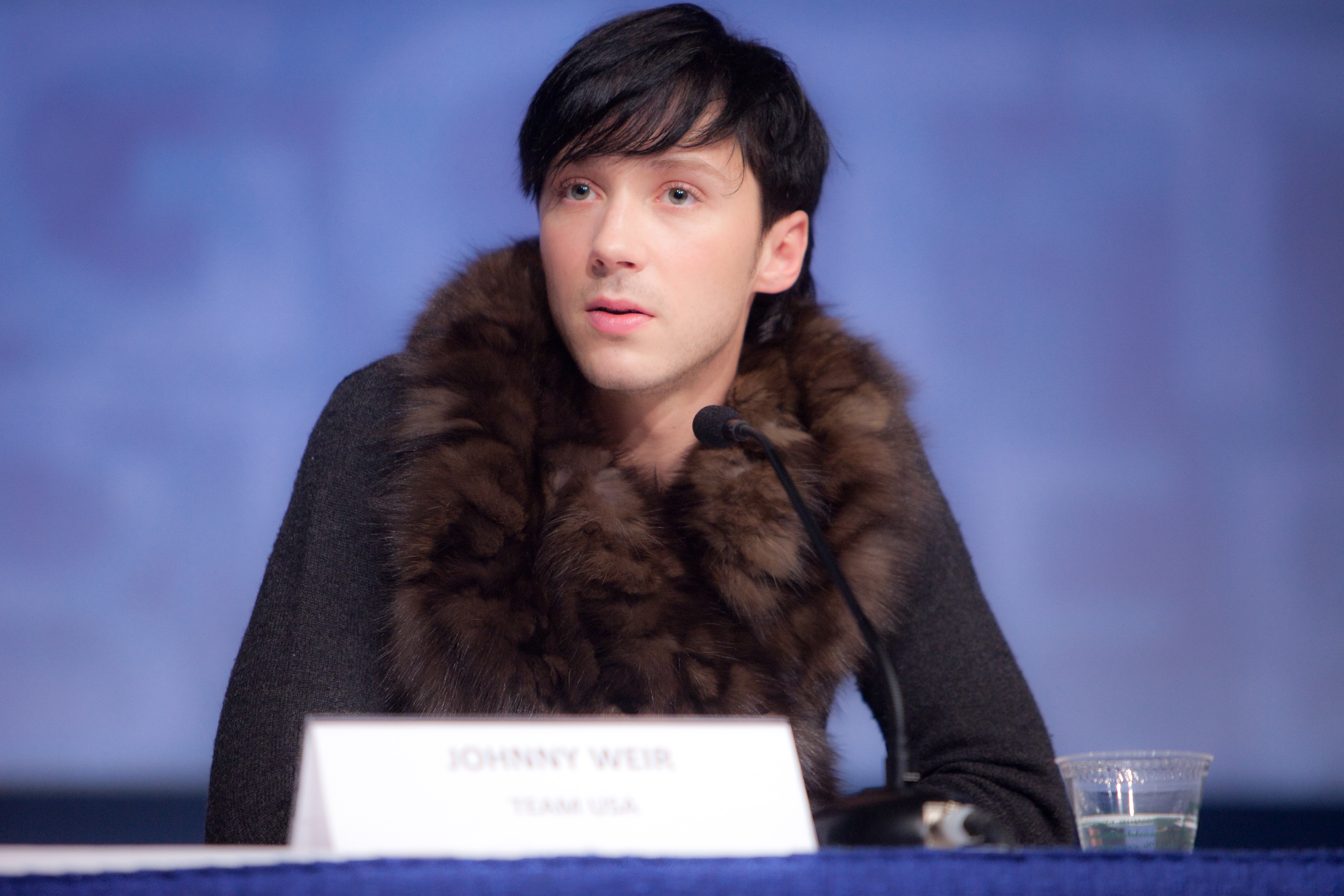In this outdoor photograph, a young man with longish, dark hair and bangs parted on one side, identified by a nametag as Johnny W.E.I.R. from Texas, USA, sits at a table covered with a blue tablecloth. Johnny, who is white and has striking blue eyes, is dressed in a dark long-sleeved shirt with a thick fur collar that drapes from his neck down to his chest. He is positioned in front of a microphone on a stand pointed toward his mouth, poised as if about to speak. His gaze is directed slightly away from the camera, and he has a serious expression. To the right of Johnny is a partially filled plastic cup of water. The backdrop behind him features a mottled purple and white curtain, adding a contrasting hue to the composition.